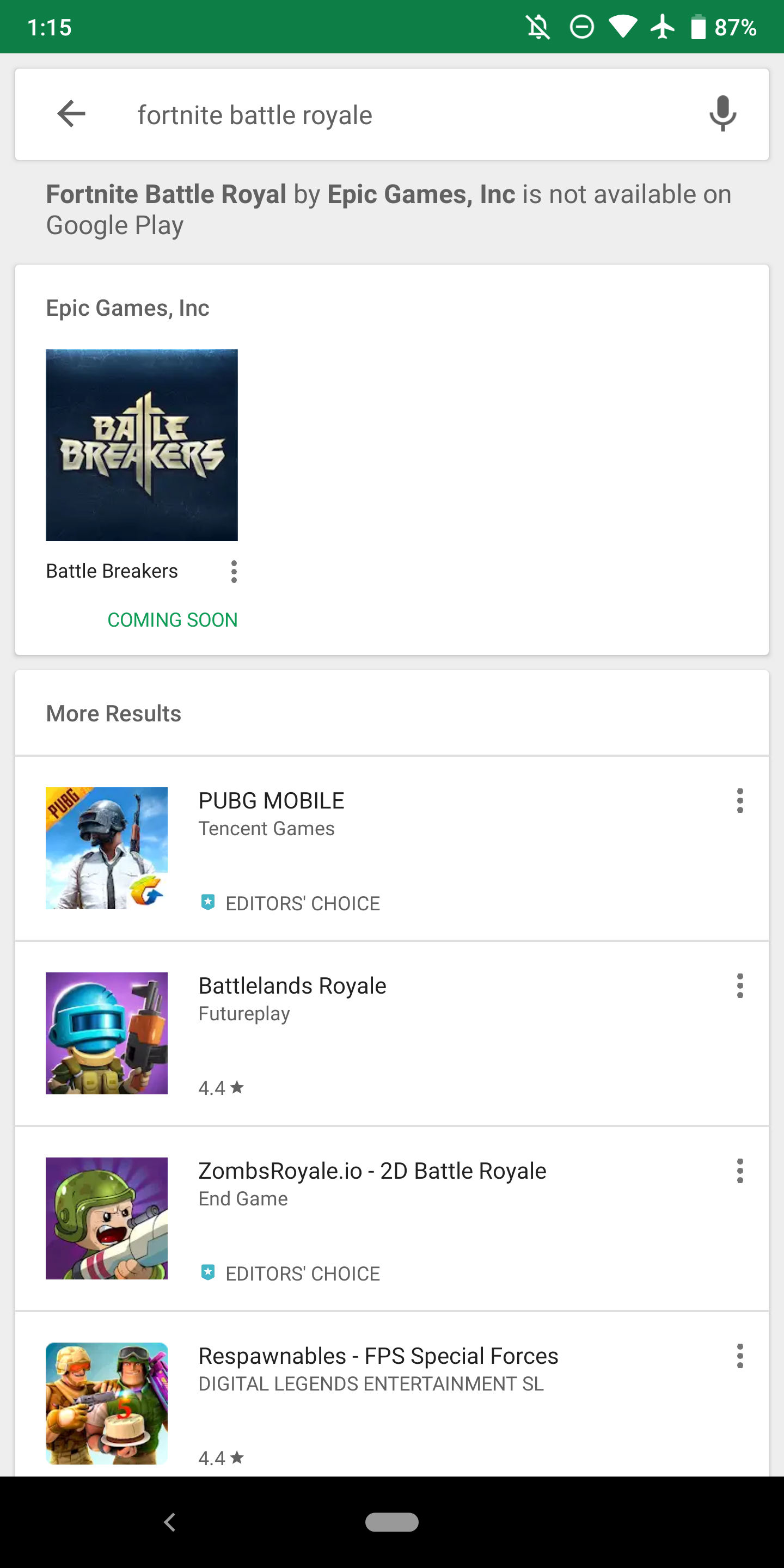The screenshot depicts a phone screen with the following details: 

At the top, the status bar features a green background with a time display showing 1:15. The notifications are turned off, and the battery is at 87%.

Below the status bar is a search bar with a microphone icon for voice input, displaying the text "Fortnite Battle Royale".

The next section of the screenshot, set against a gray background, indicates that "Fortnite Battle Royale" by Epic Games Inc. is not available on Google Play. 

Further down, there's a white rectangle containing details about Epic Games Inc., including a dark blue square labeled "Battle Breakers", which has the text "Coming Soon" beneath it.

Following this, additional search results are listed:
1. "PUBG Mobile" by Tencent Games, marked as the Editor's Choice.
2. "Battlelands Royale" by Futureplay, with a 4.4 rating (scale unspecified).
3. "ZombsRoyale.io - 2D Battle Royale" by End Game Interactive.
4. "Respawnables - FPS Special Forces" by Digital Legends Entertainment, also with a 4.4 rating (scale unspecified).